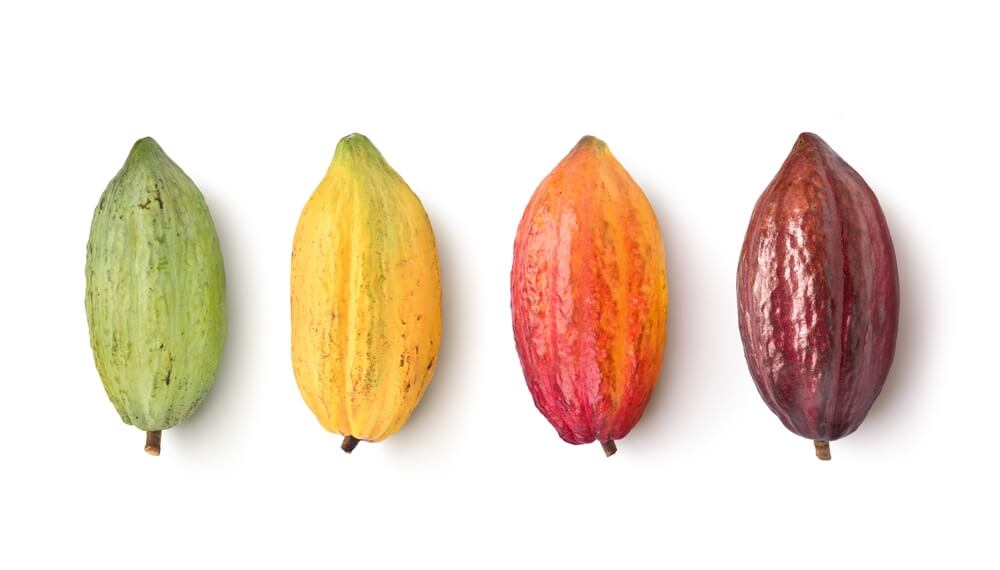This is a detailed photograph depicting the ripening stages of a particular fruit, aligned horizontally against a plain white background. The fruit, which is almond-shaped and has a small stem at the bottom, transitions through various colors as it matures. The first fruit on the left is light green, suggesting its initial stage of ripeness. To its right, the second fruit is yellow with green streaks, indicating the beginning of the ripening process. The third fruit exhibits a reddish-yellow hue, showing further ripening, while the fourth and final fruit is a deep, dark red, almost purple, suggesting it is fully ripe. All pieces display a brown skin, and the background provides no additional context, placing the focus solely on the fruit's progressive maturation.